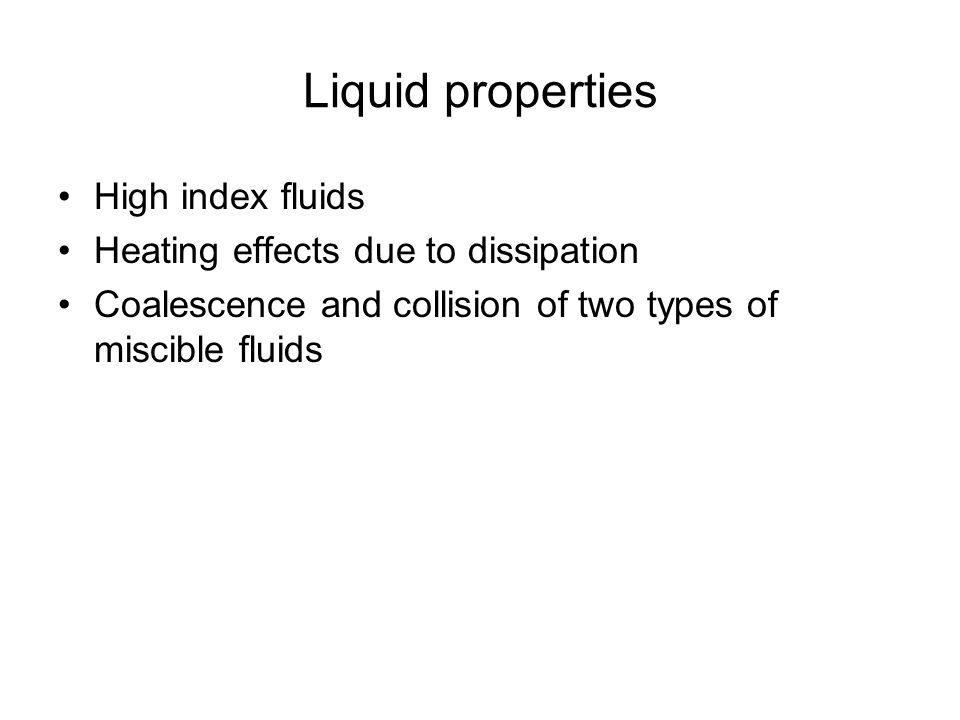The image presents a piece of text on a plain white background, resembling a slide from a business or informational presentation, possibly created using software like Microsoft PowerPoint. Centered at the top is the title "Liquid Properties" in a large, capitalized font. Below the title, three bullet points are listed in a slightly smaller, black, computer-style font, aligned to the left. The bullet points, each beginning with a capital letter, read as follows: "High index fluids", "Heating effects due to dissipation", and "Coalescence and collision of two types of miscible fluids". The text is entirely in black, without any additional images, colors, or references to websites, presenting a clean and straightforward display of the information.